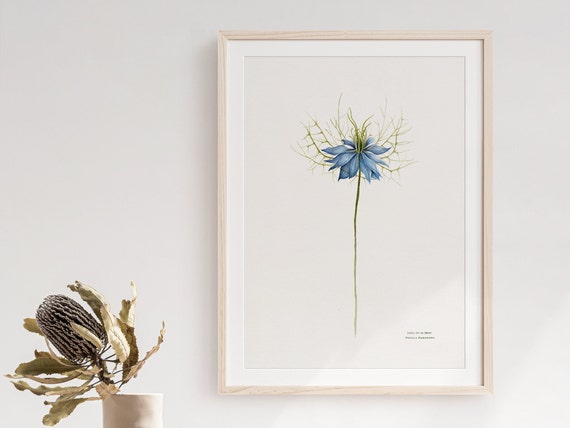The scene features a photograph of a framed artwork mounted on a white wall. The artwork itself is a detailed illustration of a blue-petaled flower with green elements, possibly stems or roots, radiating from its yellow-green center. The flower is supported by a long, thin green stem reaching towards the bottom of the image. This illustration is meticulously framed in a light tan wooden frame with a white mat border. At the bottom right corner of the artwork, there is a tiny, indecipherable, two-line text, likely the artist's name or the title of the piece.

Adjacent to the framed picture, to the left, is a dried plant set in a white or clay vase. The plant appears withered, with brown, crunchy-looking leaves, and a dark, blackish pod at its center, illustrating a theme of still life and decay. With its delicate artistic composition and subtle details, the juxtaposition of the framed flower drawing and the deteriorating real plant creates a striking visual contrast.